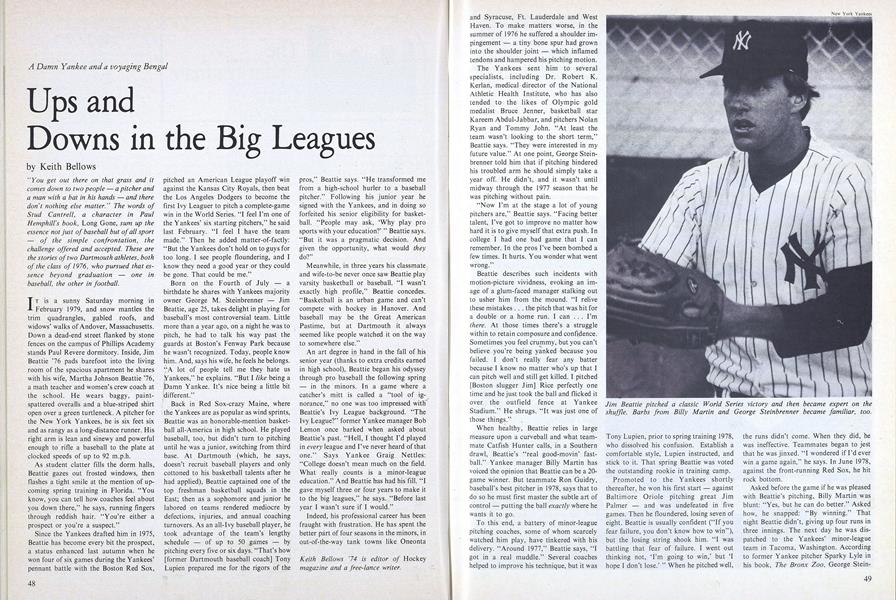This image captures an open magazine spread, pages 48 and 49, featuring an in-depth article titled "Ups and Downs in the Big Leagues" by Keith Bellows. The left page displays the article's title at the top, followed by several columns of text. The right page prominently features a black-and-white photograph occupying a large portion of the section. The photograph depicts a New York Yankees pitcher, identified as Jim Beatty, dressed in the team's classic white and black pinstripe uniform, sporting a cap with the iconic "NY" emblem. Below the image, a caption reads: "Jim Beatty pitched a classic World Series victory and then became expert on the shuffle." The backdrop of the photo reveals Beatty standing in front of a chain-link fence, holding his glove in anticipation. The article narrates the highs and lows of a major league career, encapsulating what it's like to play in the big leagues through the lens of Beatty's experiences. Additionally, a quote from an unreadable character highlights the essence of baseball, where it all boils down to the pitcher and the batter on the grass.